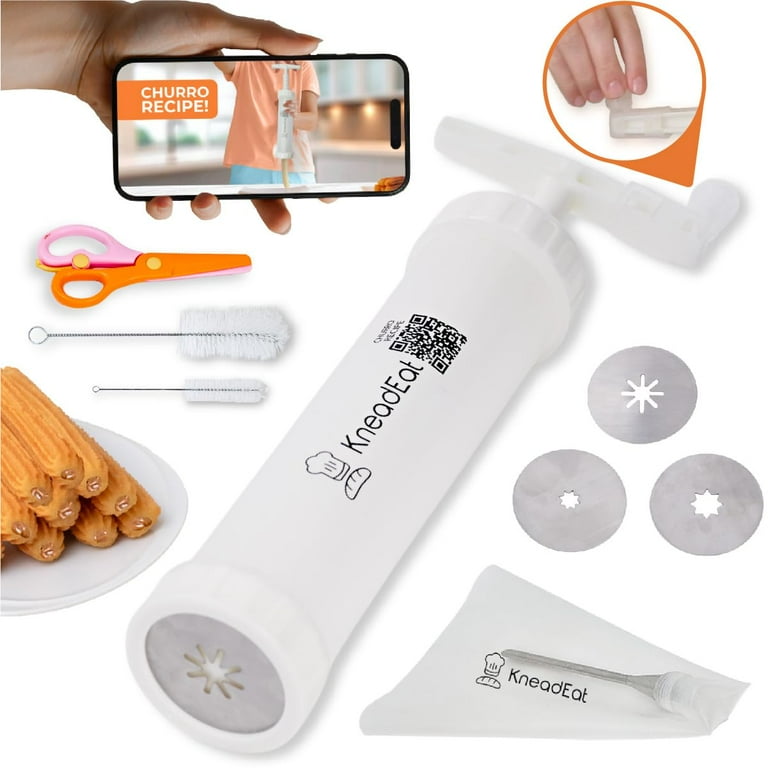The vividly staged, vertically rectangular indoor advertisement depicts the NeedEat instrument against a pristine white backdrop. Central to the image is the cylindrical, white NeedEat device, prominently featuring a handle at the top and a hole at the bottom, designed for extruding or shaping food items. The text "NeedEat" is printed in black in the center of the device, accompanied by a visible QR code labeled "churro recipe."

In the upper left corner, a Caucasian left hand is captured holding a smartphone horizontally, displaying an image of a woman in an orange shirt and blue pants using the NeedEat instrument along with the text "churro recipe." Adjacent to this, in the upper right corner, is a circle showcasing four Caucasian fingers.

Flanking the device on the right are several circular extrusion tools bearing various designs. Below these, a napkin with the "NeedEat" logo and text in black is placed, resembling a tissue paper. To the left of the NeedEat instrument lies a small pyramid of what appears to be fudge, along with pink and orange plastic scissors and two wire bottle brushes with white bristles.

This intricately detailed scene effectively highlights the functionalities of the NeedEat device, surrounded by related tools and digital enhancements, all contributing to a visually appealing and informative advertisement.